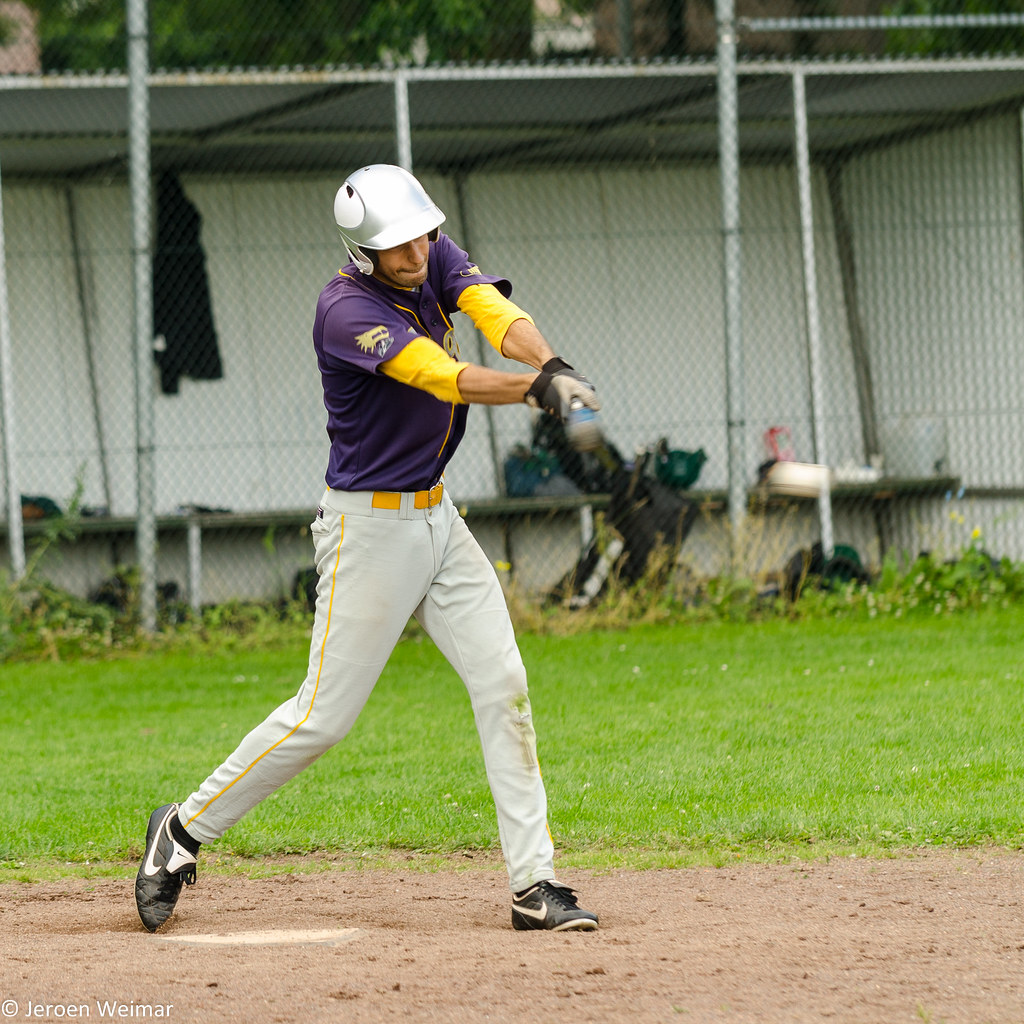This image captures a young, slender white male baseball player in mid-swing, seemingly just about to hit or having hit a blurry baseball that is about two feet behind his back, slightly lower than his bat. He is wearing a silver and white helmet, a purple jersey with yellow sleeves that extend past his elbows, and white pants accented with a yellow belt and a yellow stripe down the side. His black and white Nike shoes sport the recognizable white swoosh. The player stands on light brown dirt, with a well-maintained green grass field starting a bit behind him, sprinkled with small white flowers. In the background, we see a dugout area featuring wooden benches cluttered with various pieces of equipment, surrounded by netting. The setting appears devoid of other people, emphasizing the solitary focus on the batter. The bottom of the image bears the inscription "J-E-R-O-E-N W-E-I-M-A-R" on the left side.